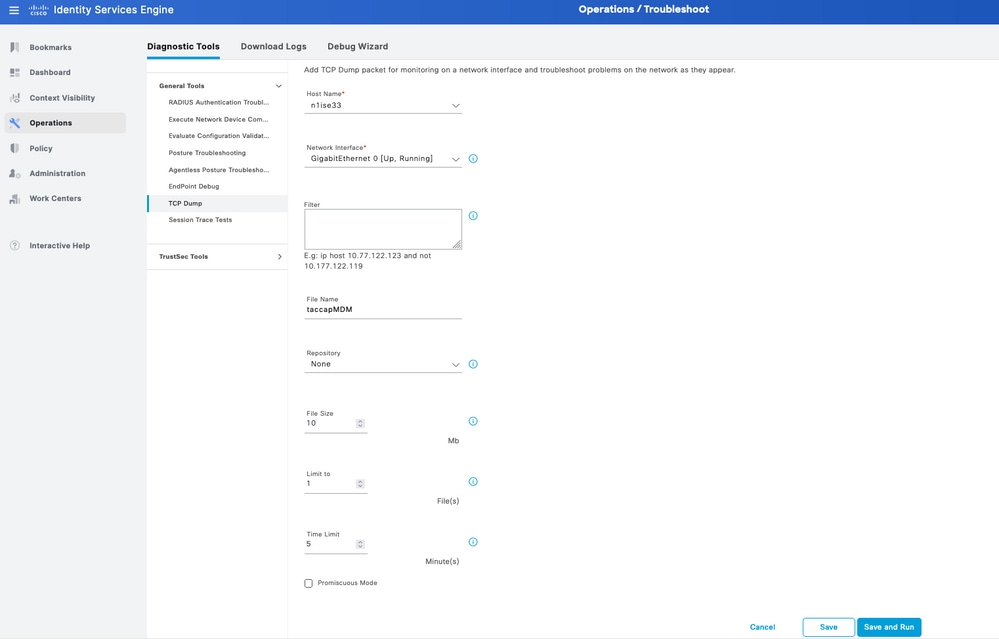This is a horizontal rectangular screenshot primarily consisting of white, with some gray and blue elements at the top. The interface belongs to Cisco's Identity Services Engine (ISE) under the "Operations / Troubleshoot" section. 

On the left-hand side, there is a navigation menu listing the following options: Bookmarks, Dashboard, Context Visibility, Operations, Policy, Administration, and Work Centers. At the bottom of this menu, there is an option for "Interactive Help" accompanied by a question mark icon.

The selected page is "Operations," which has expanded to reveal options on the right side, including Diagnostic Tools, Download Logs, and Debug Wizard. The "Diagnostic Tools" section is currently selected, displaying a list titled "General Tools." The tools listed include:

- Radius
- Authentication Trouble
- Execute Network Device
- Evaluate Configuration Validation
- Posture Troubleshooting
- Agentless Posture Troubleshooting
- Endpoint Debug
- TCP Dump
- Session Trace Tests
- Trust-C Tools

Within this list, the "TCP Dump" tool is selected. This section allows the user to fill out various fields such as Host Name, Network Interface, Filter, File Name, Repository, File Size Limit, and Time Limit. At the bottom, there are three action buttons: "Save & Run," "Save," and "Cancel."